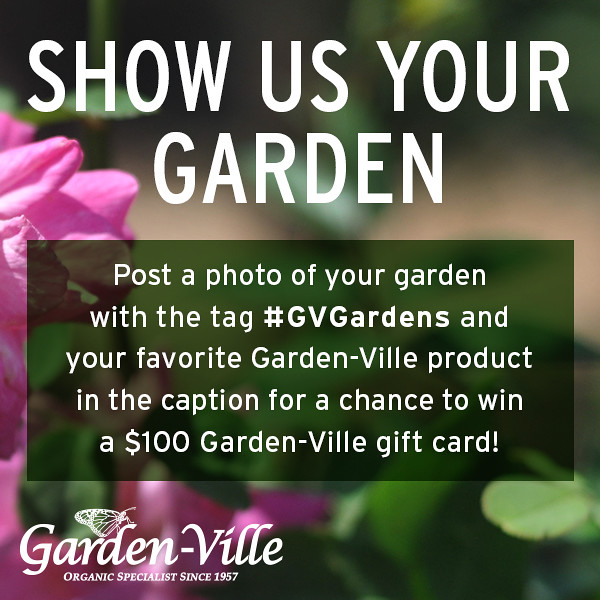The image is a vibrant advertisement with a blurred background that features pink flowers on the left and green leaves on the right. At the top, the phrase "Show us your garden" is prominently displayed in bold, white capital letters. Below this, inside a transparent black box in white font, it invites viewers to "Post a photo of your garden with the tag #GVGardens and your favorite Gardenville product in the caption for a chance to win a $100 Gardenville gift card." Towards the bottom left of the image, the logo "Gardenville" is shown in bold white font, with the words "Organic Specialist since 1957" beneath it in unbolded white font. Adding a whimsical touch, a white butterfly stencil is delicately perched on the letter 'D' in "Gardenville." The setting appears to be outdoors, bathed in natural daylight, emphasizing a garden-like environment. The overall color palette includes white, black, green, pink, and a touch of brown, gray, and tan, enhancing the inviting and organic feel of the advertisement.